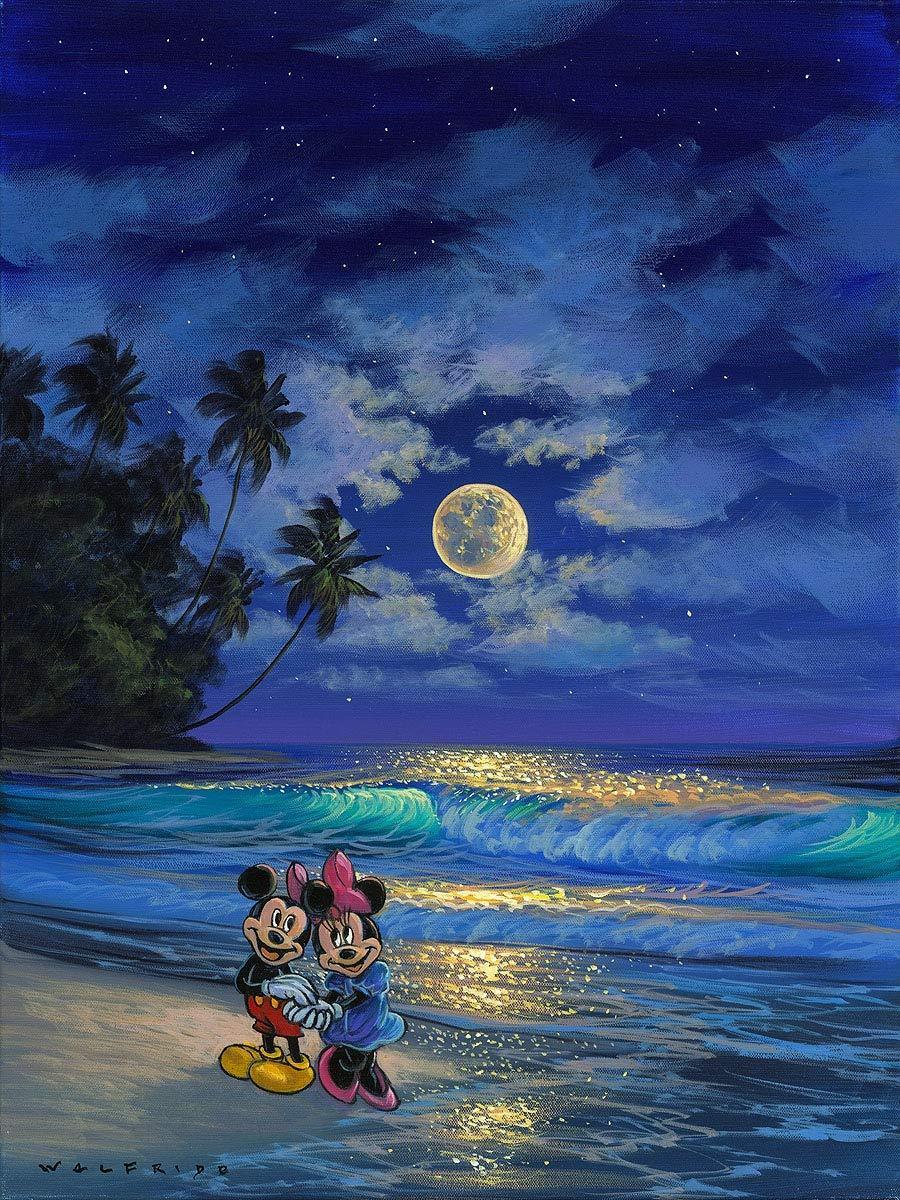This detailed Disney illustration showcases Mickey and Minnie Mouse on a tropical beach at night. The scene is bathed in a dark blue sky with overcast clouds, allowing stars and a large glowing moon to peek through. A setting sun also adds to the dusky ambiance. Gentle waves crash against the shore, accentuating the serene setting. On the left, tall, thin-trunked palm trees lean out over the water, seemingly windblown from the ocean breeze. In the foreground, Mickey, wearing his iconic red shorts and yellow shoes, and Minnie, adorned in a blue dress with a pink bow and pink shoes, hold hands and smile lovingly at each other. Positioned at the bottom left of the canvas, the texture of which is visible, adding depth to the painting, is a black signature reading "W4LFRIDO." This meticulous artwork conveys a romantic and tranquil atmosphere, encapsulating a tender Disney moment amidst a tropical paradise.